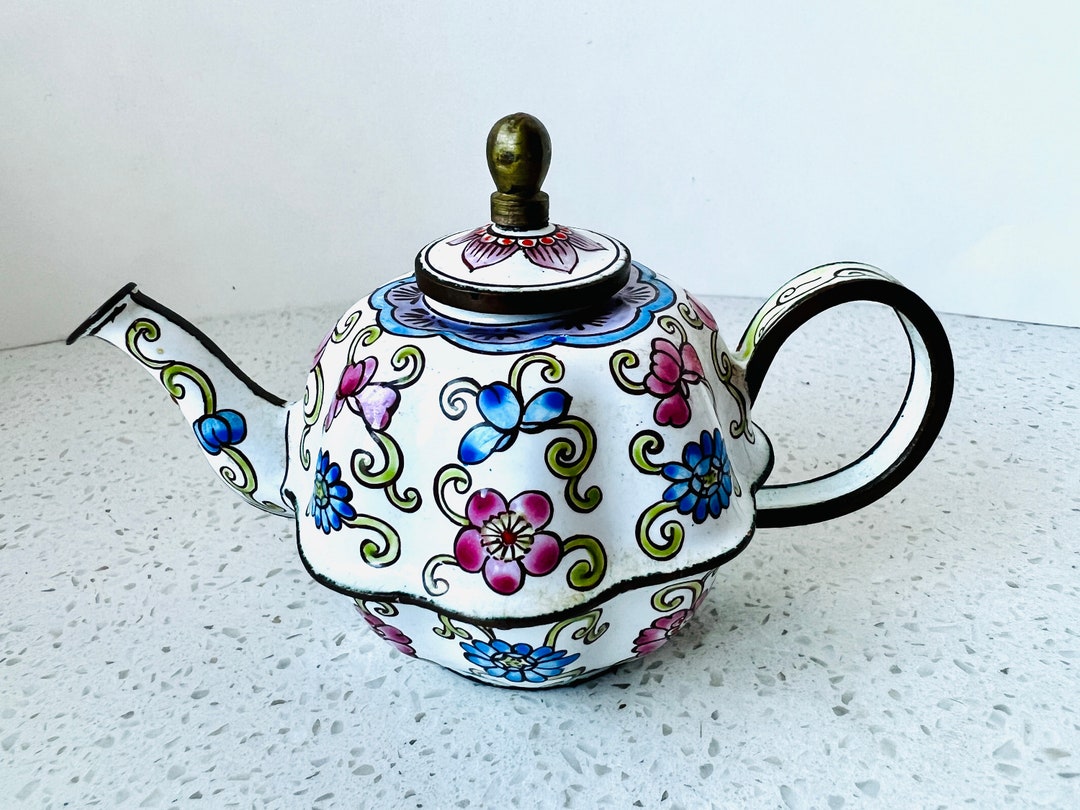This photograph showcases a highly decorative and colorful teapot resting on a white granite countertop with gray flecks. The white wall behind provides a stark contrast to the vibrant teapot. The teapot itself features an eye-catching bright pink, blue, and purple floral design, with large blossoms and green tendrils spread across its surface. Intricate black lines outline the pouring spout and the ribbon-like handle, both of which are detailed with smaller flower buds and vine patterns. The teapot shape is slightly irregular, with the bottom appearing smaller and somewhat tucked in, possibly bordered by a black ledge. The lid, resembling a flower's petals, has a distinctive black handle, further adorned with a copper attachment. The overall design is a whimsical blend of colors and patterns, making the teapot a striking centerpiece on the countertop.